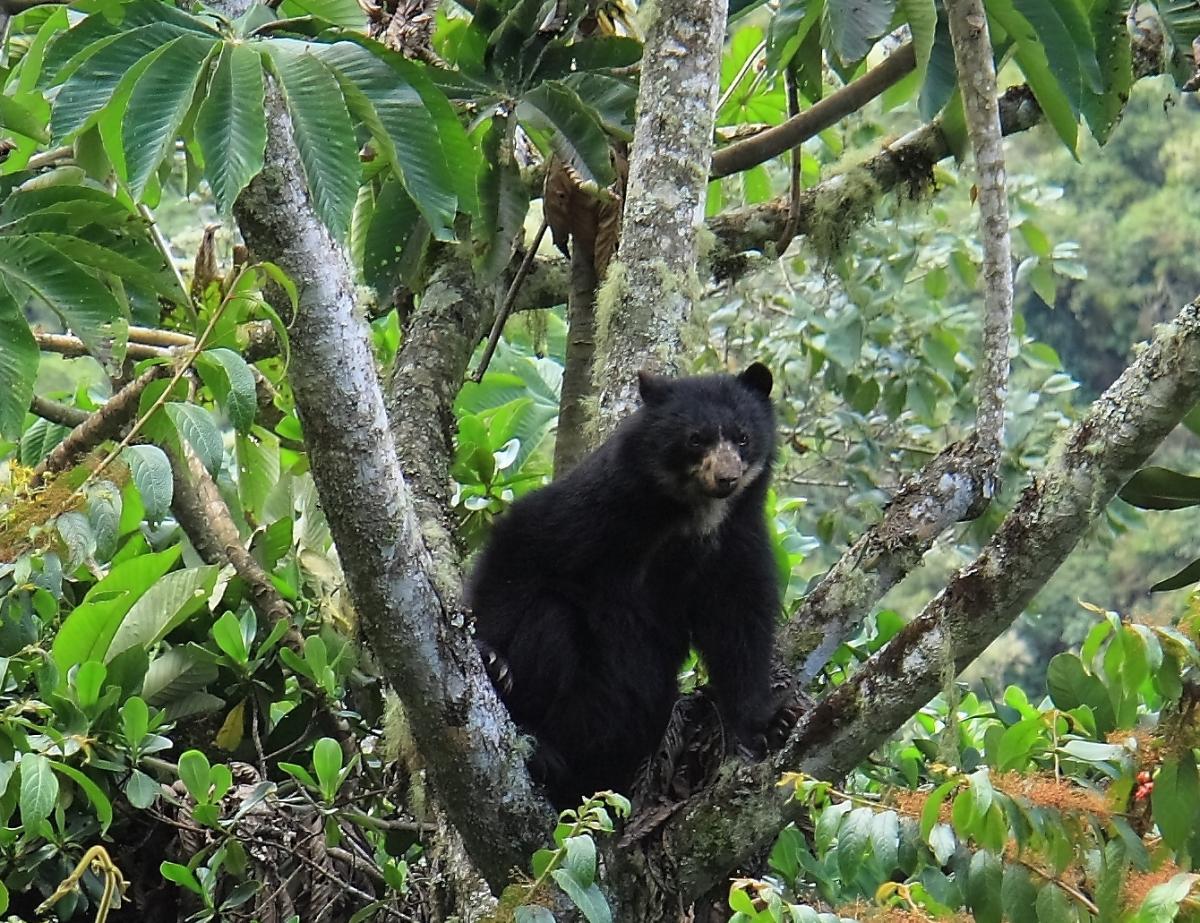This is a daytime color photograph of a black bear perched in the center of a large tree within a dense, tropical forest. The black bear is balancing on the larger limbs that branch out from the trunk, creating a round spot where the bear sits. The bear is facing straight ahead with its two front legs spread out for balance, one paw resting on a branch to the right and the other paw on a branch to the left. The bear's body is predominantly black with a distinct brown diamond-shaped marking around its nose, between its eyes, and extending under its neck. The tree is surrounded by long, slender palm leaves and dense greenery, emphasizing the tropical environment. The image captures the lush foliage and extensive tree canopy that frame the black bear against the vibrant forest backdrop.